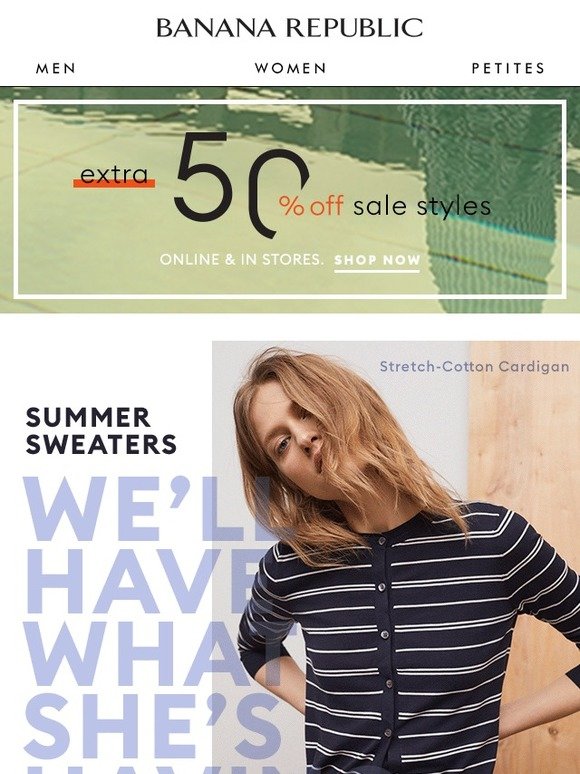This image is a screenshot of the Banana Republic website. At the top of the screenshot, the website's header has a white background with "Banana Republic" displayed in black font at the center. The navigation links are positioned on either side: "Men" on the left, "Women" directly beneath the "Banana Republic" logo in the center, and "Petites" on the right.

Below the header, there is a large rectangular banner with a grayish background that advertises an "Extra 50% Off Sale Styles," featuring a hint of what appears to be a green sweater on the right.

In the lower right-hand corner of the screenshot, there is a photograph of a young woman, likely in her early 20s, with dark blonde, shoulder-length hair covering part of her face. She has her head turned and slightly cocked to one side. She is modeling a black sweater adorned with small horizontal stripes and white buttons down the front. To the left of the photo, on a white background, the text "Summer Sweaters" is written in black font. Beneath this, in light lavender-colored font, it reads "we'll have what she's...," with the remaining part of the website cut off at the bottom of the image.